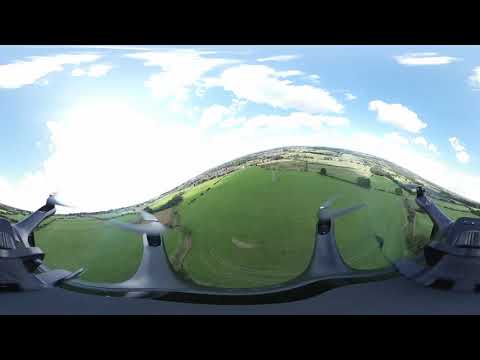The image is a highly detailed 360-degree panorama captured from a quadcopter drone hovering approximately 100 to 200 feet above a vast, green countryside. The perspective, enhanced by a fisheye lens, gives the impression of the viewer looking down from atop a windmill or a high vantage point. It showcases an expansive landscape below, filled with lush green fields, interspersed with cornfields, trails, and some dividing trees marking property lines. Scattered houses and buildings can be seen in the distance, making the transition from rural to urban almost seamless. The sky above is a clear blue, adorned with fluffy white clouds, and brilliantly lit by the midday sun, casting a bright glow over the entire scene. In the foreground, the gray quadcopter drone with its four visible rotors dominates the bottom of the image, adding a modern technological touch to the otherwise serene, pastoral view. High up in the sky and on top of the windmill-like structure, a small bird perches, adding a touch of life to this tranquil yet dynamic scene.